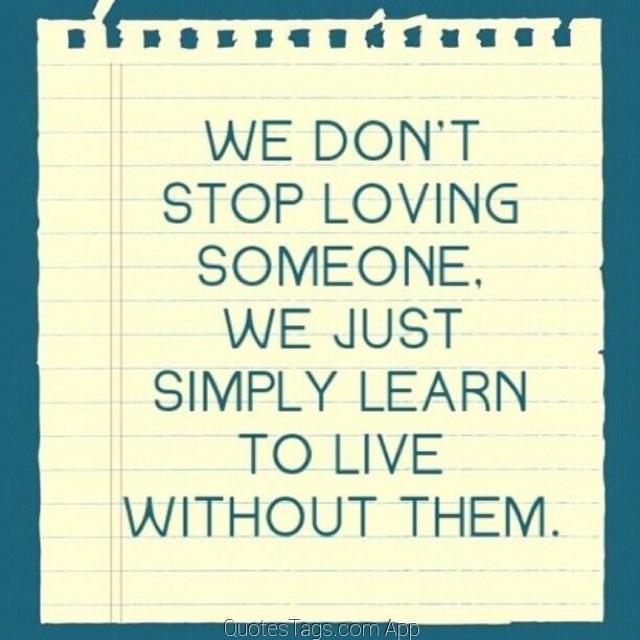This digitally created meme features a teal blue background with an image of a yellow piece of notebook paper that has blue lines and appears to be torn from a spiral notebook at the top. The primary focus of the image is the text, which reads "We don't stop loving someone, we just simply learn to live without them," written in teal capital letters spread across seven lines from top to bottom. At the bottom of the paper, in small print, is the attribution "QuotesTags.com App." The overall color palette of the meme includes teal, yellow, and blue, and the entire design emphasizes a minimalistic yet impactful presentation of the quote.